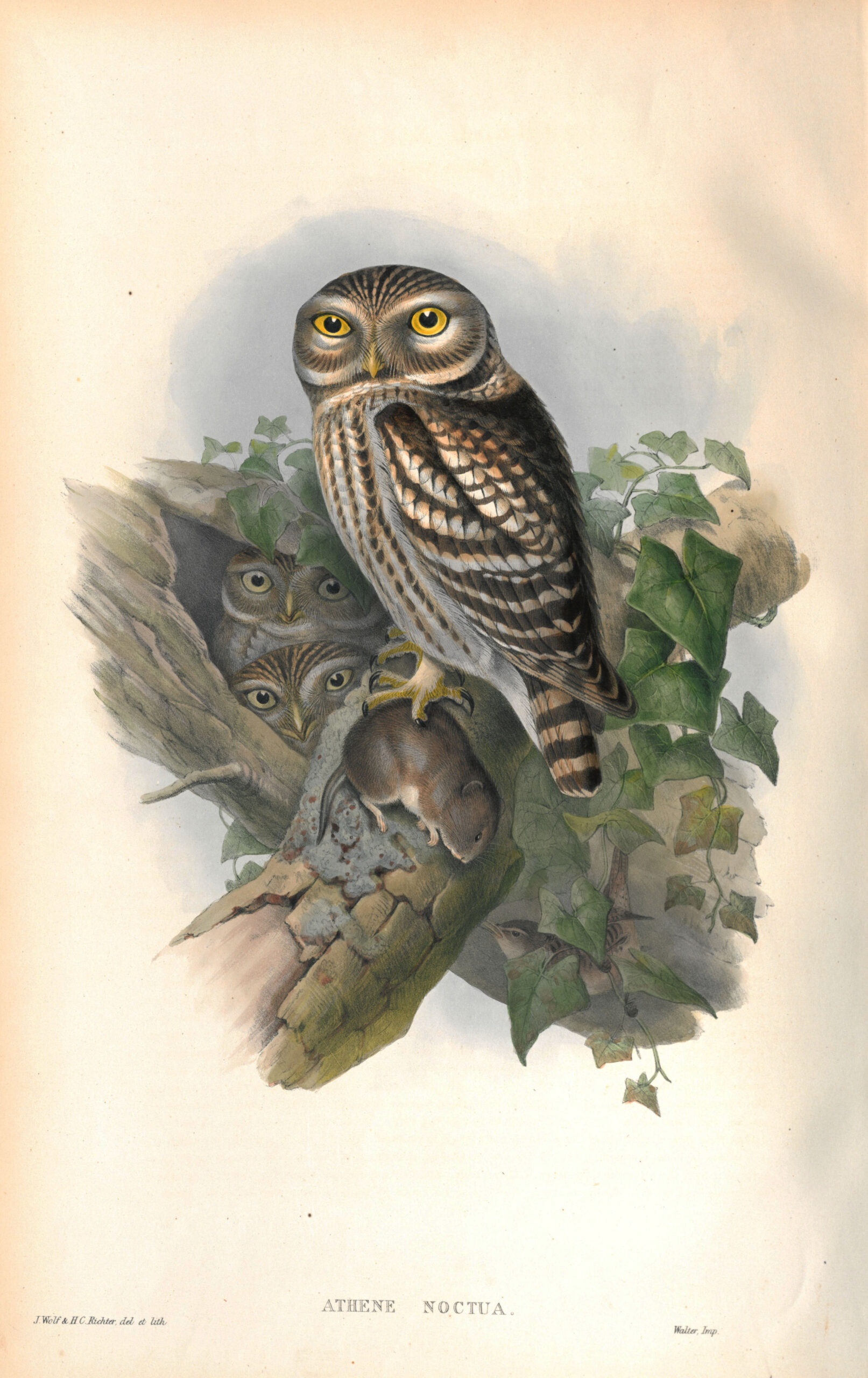The image is a vintage, vertically oriented illustration resembling a page from an old botanical reference book. It prominently features a mother owl, identified as Athene noctua, perched on a tree limb partially covered with angular, heart-shaped green foliage and spiraling ivy. The owl grips a captured rodent in her talons, poised to feed her two baby owls peeking out from a nest nestled within a crevice in the tree limb. Both the mother and baby owls are meticulously colored in hues of brown and gray, with striking golden eyes and black pupils. In the background, a blue hue fades into an off-white, adding depth to the artwork. Notably, there appears to be another bird, similar in coloration but possibly of a different species, partially hidden behind the leaves. Below the main illustration, the text reads "Athene Noctua," accompanied by additional smaller text, including "J. Wolf and H.C. Richter et al." The overall composition is richly detailed and evokes the character of classic ornithological plates.